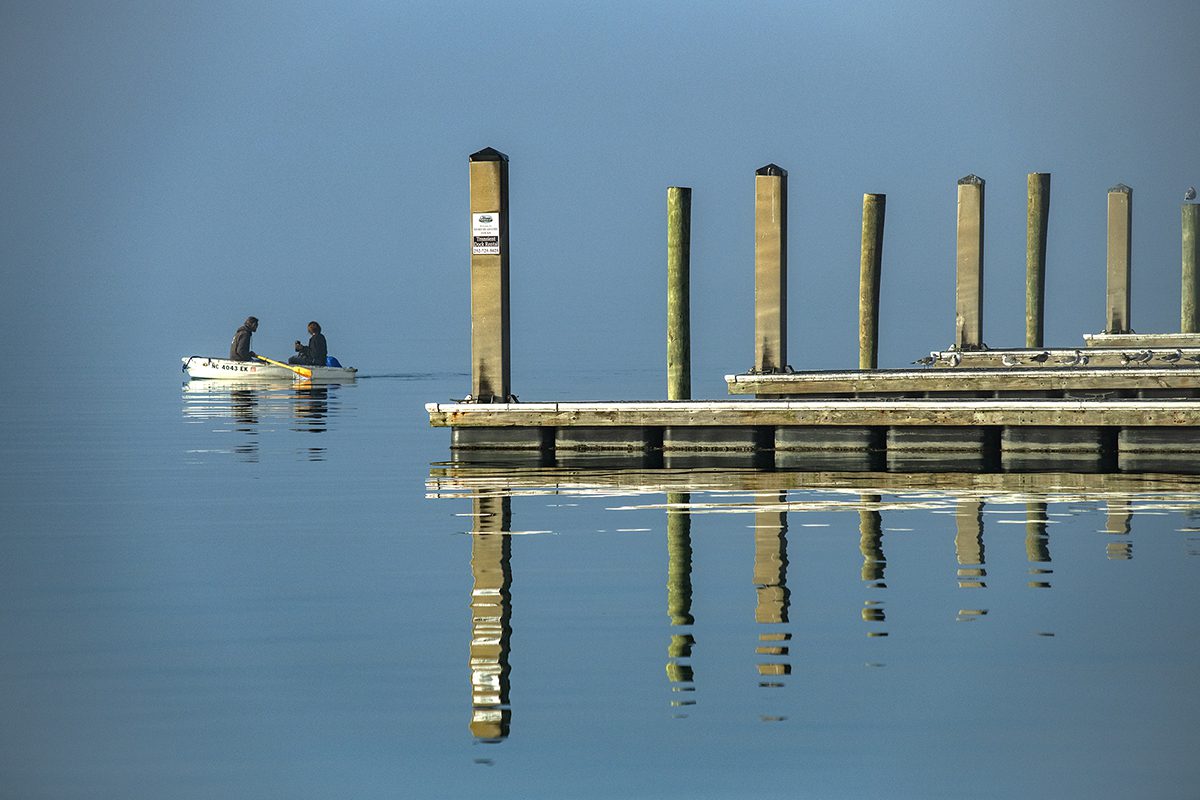This digital art image captures an angled, serene scene of a deep blue lake blending seamlessly with a pastel blue sky, creating a hazy, tranquil ambiance. Dominating the left side, there's a small white wooden rowboat with the identification "WC 4043EX," containing two men facing each other. One man dips vibrant yellow paddles into the calm water. To the right, a line of approximately four aged wooden docks, their light brown color muted by time, extends into the water. Reflecting off the tranquil surface, these docks are characterized by alternating thick boxy and thinner round poles, with some steps leading up. One of the poles features an unreadable white sign. Altogether, the scene exudes a peaceful atmosphere with the docks and boat cohesively complimenting the natural beauty of the lake.